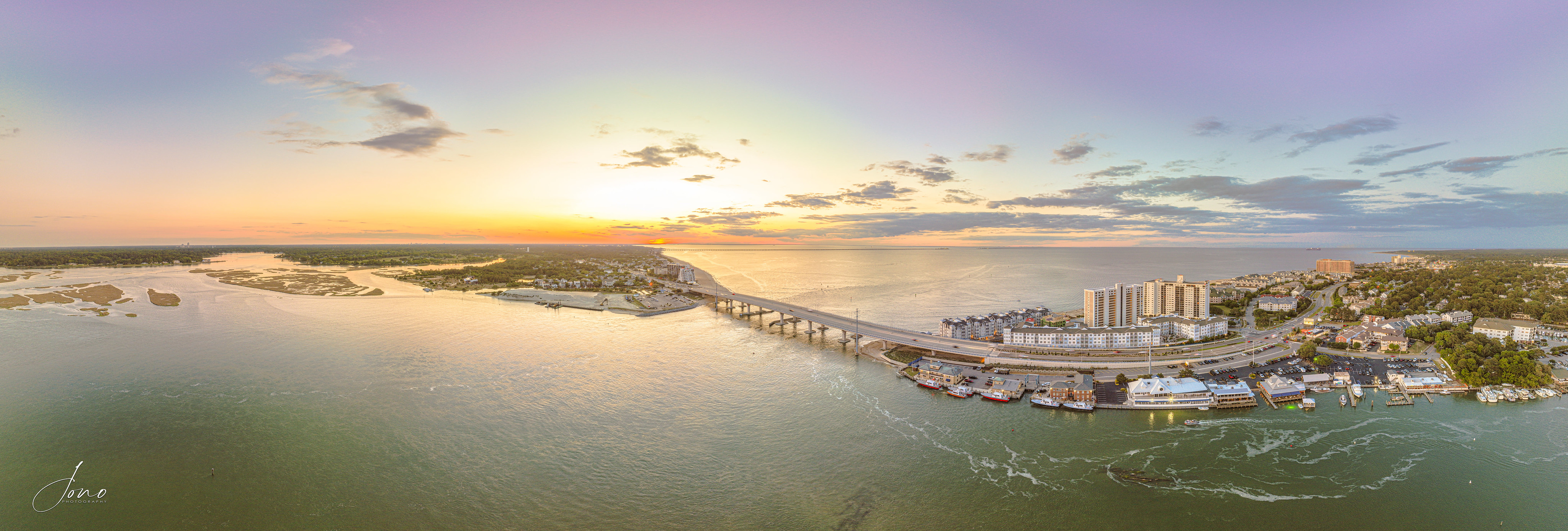The image captures a breathtaking aerial view of a coastal city during the golden hour of either sunrise or sunset. On the right side, the cityscape features a mix of tall high-rise buildings and modest-sized structures, complemented by shorter buildings along the bustling waterfront. The skyline is painted with a blend of blue, orange, and yellow hues, suggesting the sun is just above the horizon. Dotted with a few light gray clouds, the sky adds to the serene atmosphere. Stretching across a vast, bluish-green body of water, a long bridge connects the vibrant city to a tranquil, largely undeveloped expanse of land, possibly an island or a peninsula, characterized by lush forests and greenery. The water below the bridge appears calm with gentle waves. Several boats are visibly moored along the shoreline, enhancing the waterfront’s charm. In the lower left-hand corner of the image, the word "JONO" is subtly inscribed.